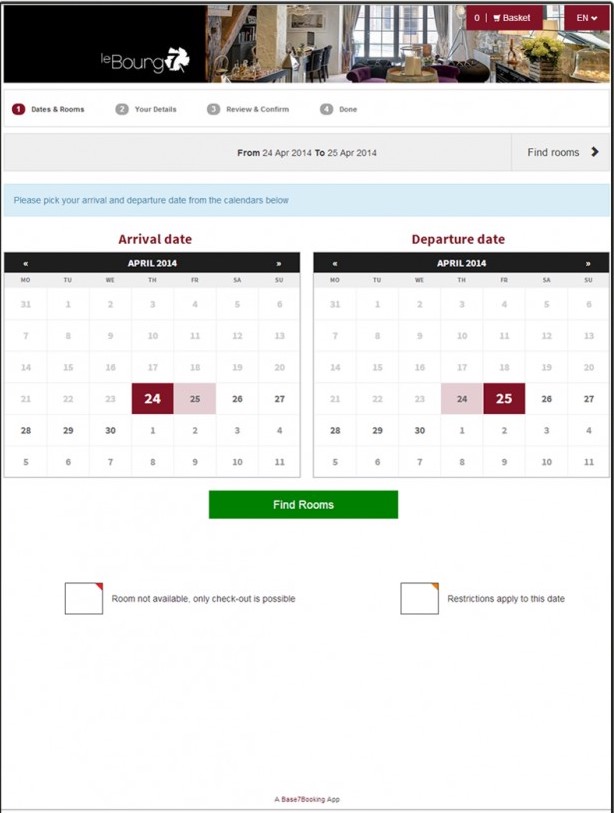The image features a white background with a prominent heading at the top that reads "Le Bong 7." Below the heading, there is an elegant photograph of a luxurious room with large windows, comfortable couches, and chairs, exuding a sense of coziness and sophistication.

At the top of the image, there are two red buttons. The first button is labeled "Basket," and the second button says "In." Adjacent to these buttons is a white box that has a red circle with the number "1" inside it, indicating a step in a multi-step process. The text next to the box reads "Dates and Rooms." Below this are additional steps numbered within red circles - "2" for "Your Details and Services," and "3" for "Cost and Done."

Additionally, there is a blue box specifying the date range from "24th April 2014 to 25th April 2014" with a "Find Rooms" button and a right arrow attached. Another blue box instructs users to "Please pick your arrival and departure date from the options below."

Two calendars are displayed for selecting arrival and departure dates. The calendar for departure dates has the 24th of April highlighted in red, while the departure date calendar highlights the 25th of April in a red box. Below these calendars, a large green button labeled "Find Rooms" is prominently displayed.

In the lower section, a small box with the top right corner in red signifies "Room Not Available, Only Checkout Possible." Another adjacent square with a red top right corner indicates "Restrictions Apply to the Date." At the very bottom, there is an unreadable line of small print text.